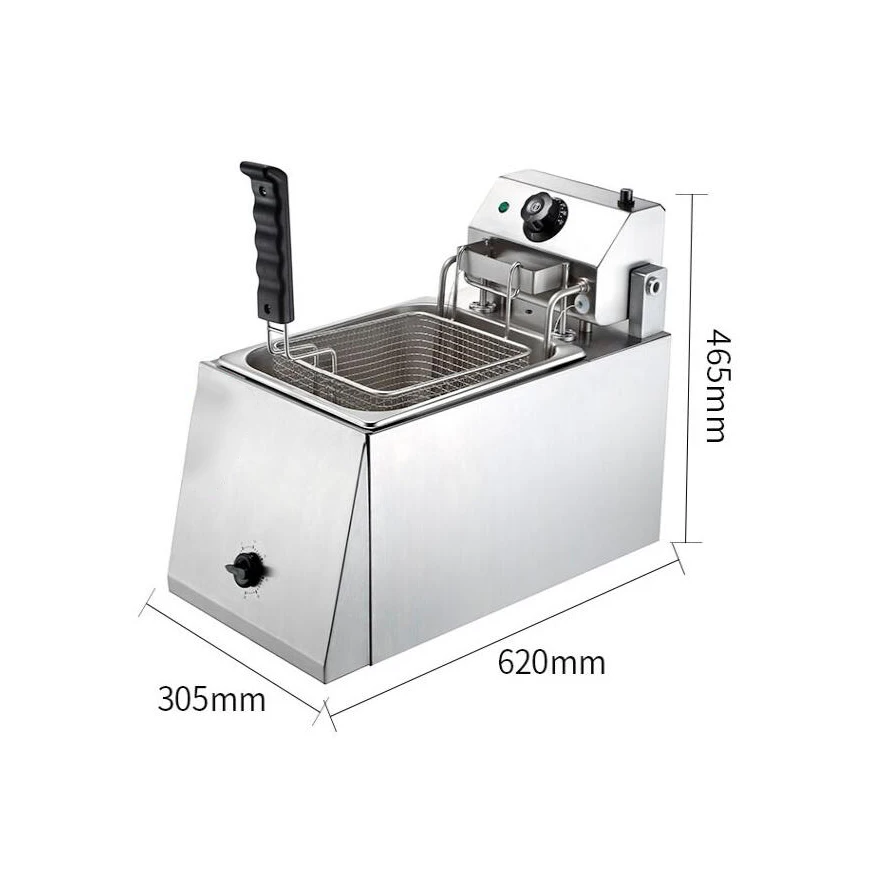The image showcases a sleek, stainless steel deep fryer, meticulously positioned on a flat white surface against an unobtrusive white background, creating the impression that it is suspended in a pristine, empty void. Detailed measurements encircle the fryer, indicating its dimensions: 465 millimeters in height, 620 millimeters in length, and 305 millimeters in width. The deep fryer features smooth sides and a user-friendly black plastic knob adorned with various numbers and notches on the front. 

At the top, a receptacle holds a robust, black-handled metal basket designed for easy food insertion and retrieval. This is complemented by an upper raised area with another black knob and a small green LED light. The back of the fryer houses essential equipment, including the control knobs and a button for cleaning access. Two heating element rods protrude from the front, extending into the oil compartment to ensure the oil heats efficiently. This comprehensive design demonstrates not only the fryer’s dimensions and materials but also its functional components, all aimed at delivering a reliable and safe cooking experience.